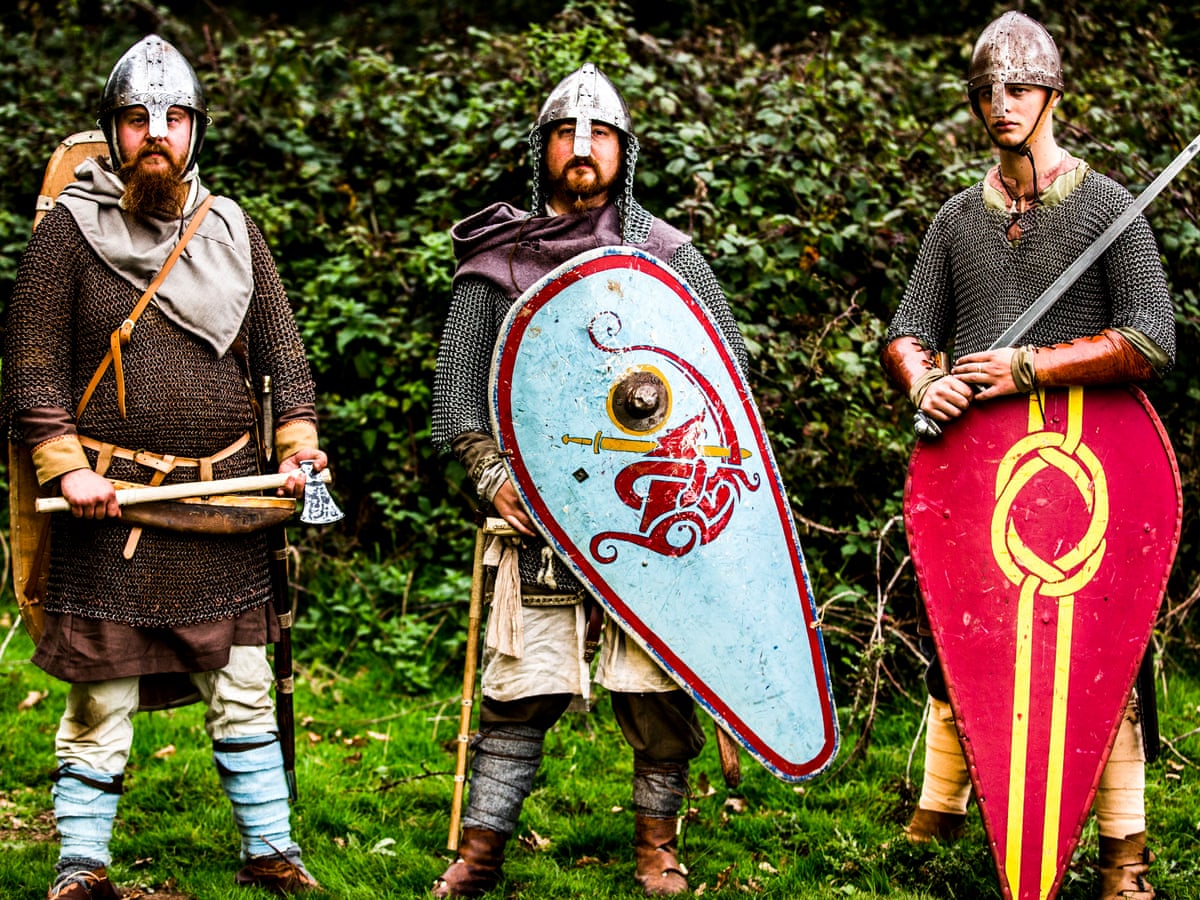In the detailed image, three men are depicted as medieval knights, possibly for a reenactment or cosplay event, standing on bright green grass with a backdrop of dark green shrubbery. All of them wear pointed steel helmets with nasal guards. The man on the left, slightly chubbier with a beard, dons mid-thigh length brownish chainmail over a brown tunic and a gray scarf. He holds a small axe and has a shield strapped to his back. His legs are wrapped in white and light blue leggings, and he wears dark brown shoes.

The man in the center, also bearded, sports chainmail over a cream tunic and a slightly purplish cowl. His shield, held in front, is predominantly white with an intricate red and yellow pattern and a red border. Though his weapon isn't visible, it may be attached to his leg or hip. He completes his outfit with grey socks and brown shoes.

The younger, clean-shaven man on the right wears chainmail and a metal helmet with a nose piece. He holds a sword against his body and carries a large red shield with a yellow knot emblem. His attire includes brown leather arm guards and brown shoes.

All three show serious expressions, emphasizing their dedication to accurately portraying their medieval roles.